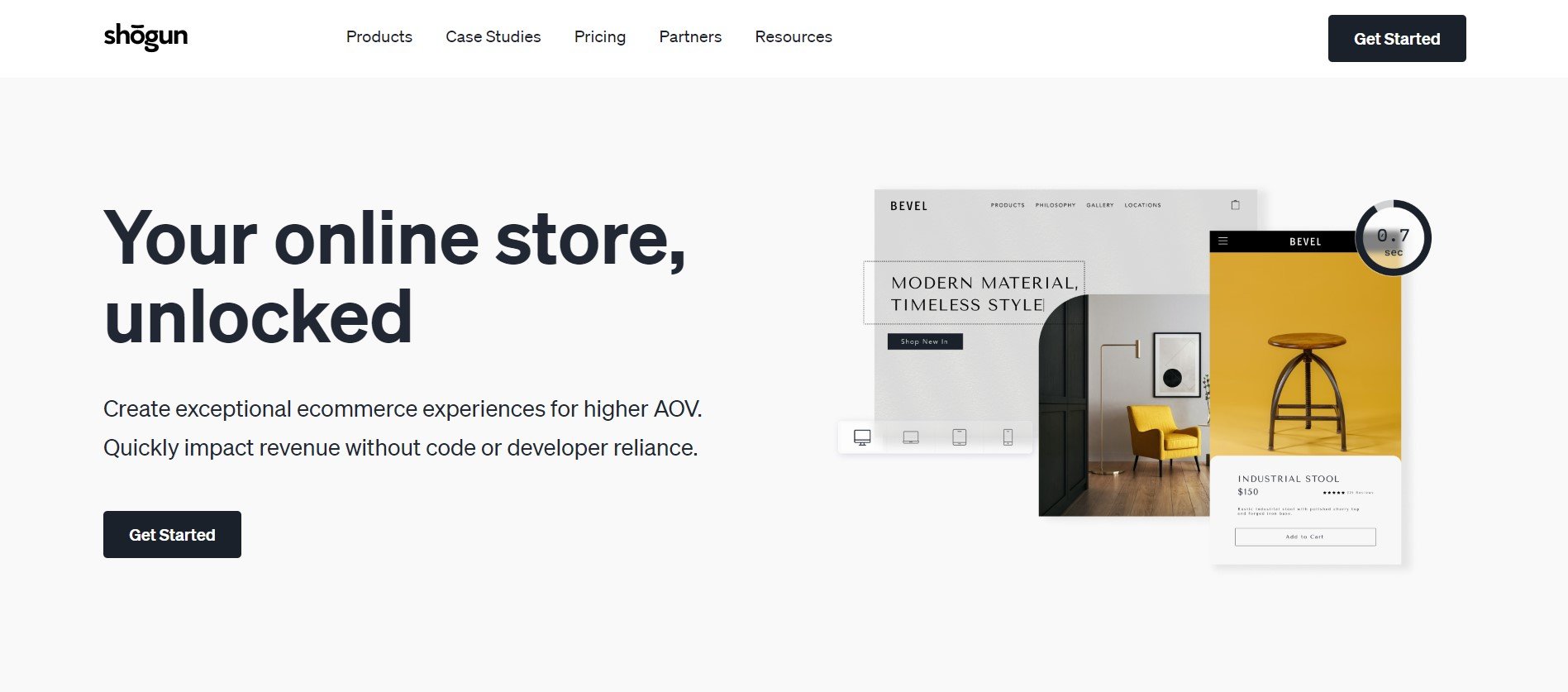A detailed screenshot depicts a webpage from a website named "Shogun." The logo is a minimalist text design, set in black heavy font in lowercase, with a down-pointing arrow above the "O." To the right of this logo, there is a horizontal navigation menu that includes the following items: Products, Case Studies, Pricing, Partners, and Resources. At the far right end of the menu, there is a call-to-action button labeled "Get Started."

The layout appears to be a hero section of the page, with large, bold Helvetica text on the left that reads, "Your online store, unlocked." Following this headline, two lines of supporting text are displayed: "Create exceptional e-commerce experiences for high AOV. Quickly impact revenue without code or developer reliance." Below this text is another "Get Started" button.

To the right side of the hero section, there are three overlaid images. The background image displays a placeholder for a sample website labeled "Modern Material, Timeless Styles, OC Revel." Overlaying this is a photograph of a simple chair situated on a wooden floor, accompanied by a lamp and some wall art. Adding another layer, a screenshot from a mobile phone is displayed, highlighting the same "Revel" or "Revel" theme. This mobile interface shows an old-fashioned industrial stool with a round seat and four metal legs. The stool features a central screw for height adjustment. Above the product image is a progress or loading bar within a circle, indicating a fill level close to 90%, with the number "0.7" partially visible. Below this, the text "industrial stool" is displayed along with options to purchase the item.

Overall, the webpage appears to be a template or sample for an online store, showcasing how the platform can be used to create visually appealing and functional e-commerce sites.